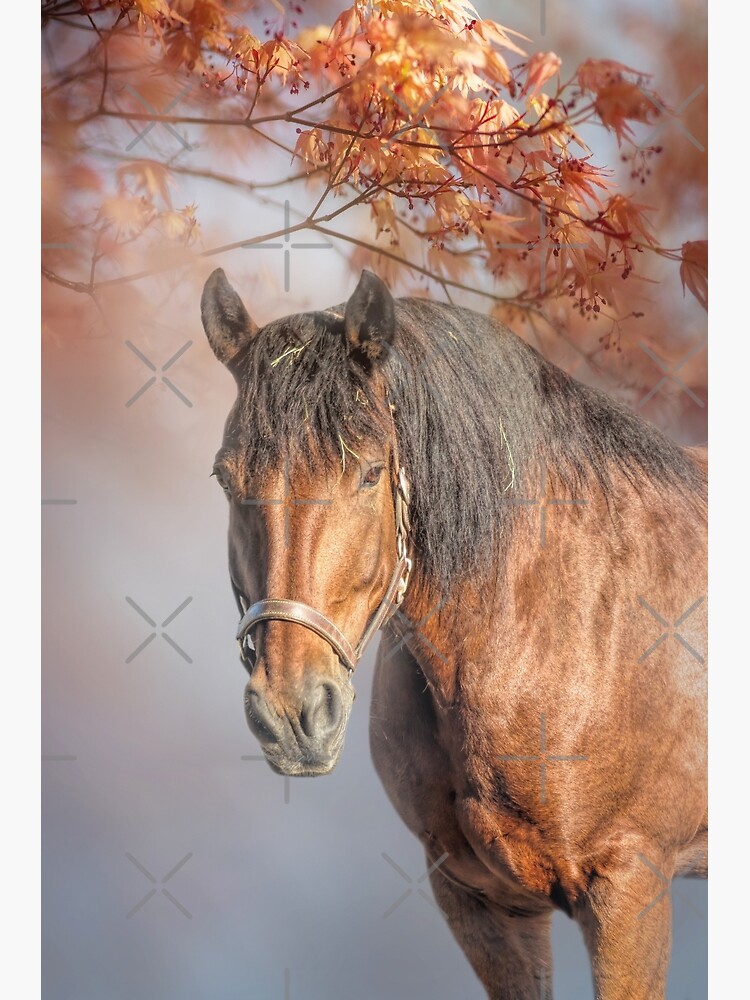A beautifully illustrated horse stands under a tree with orange-yellow flowers and reddish berries. The horse, with a shiny chestnut or roan coat, faces slightly to the side, its head positioned near the center-left of the image. Its dark brown body contrasts with a black mane that adorns the top of its head, extends down the top of its back, and accentuates its black snout. A brown leather bridle, detailed with gray hardware, wraps around its face. The background is artistically blurred, featuring hues of dark blue, dark orange, and light gray, making the horse and the tree stand out prominently. Small strands of hay are caught in the horse's mane and forelock, adding a touch of rustic charm to the scene.